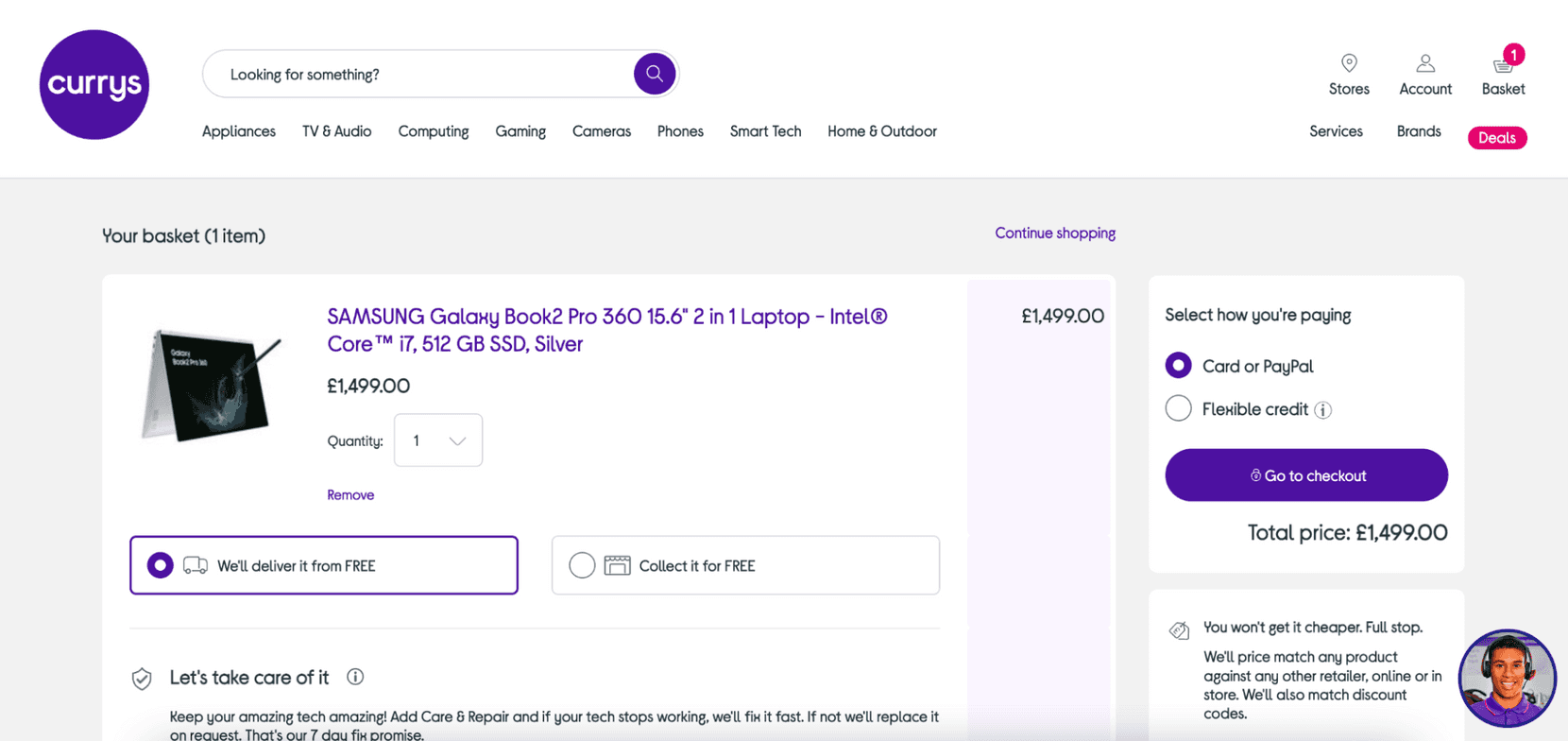The image is a screenshot from an e-commerce website, specifically the shopping cart page. At the top left corner of the page is the company's logo, "C-U-R-R-Y-S," written in white lowercase letters centered within a purple circle. The background of the page is predominantly white.

Below the company logo, there is a horizontal navigation menu. The categories listed from left to right include: Appliances, TV & Audio, Computing, Gaming, Cameras, Phones, Smart Tech, and Home & Outdoor. Above this menu, a large white search box is prominently displayed.

On the top right corner of the page, there are several icons and elements aligned from left to right: a basket icon with a small red circle containing the number "1," indicating there is one item in the cart; an account label next to an icon representing the user account; and a stores label.

The main section of the shopping cart page features a light lavender background. In the forefront, there is a large white rectangle displaying the product details. The product listed is a "Samsung Galaxy Book II Pro, 360, 15.6 inch, two-in-one laptop, Intel Core i7, 512GB SSD Silver," written in the same purple color as the company's logo. The price of the item is £1,499.00, and the quantity specified is one. Beneath these details, it states "We'll deliver it for free," also in purple text.

To the right of the product details, there is a white square box labeled "Select how you're paying." The available payment options, including Card or PayPal, have been selected by the user. Below this box is a purple button with rounded edges that says "Go to checkout" in white text. Lastly, the total price of the items in the cart is reiterated as £1,499.00.

In the lower right-hand corner of the page, there is a photo of a likely customer service representative within a round circle. The representative is wearing a purple shirt that matches the company’s color theme and a headset, suggesting he is there for customer support. He has dark hair, a friendly smile, and possibly hails from an Italian or Middle Eastern background.